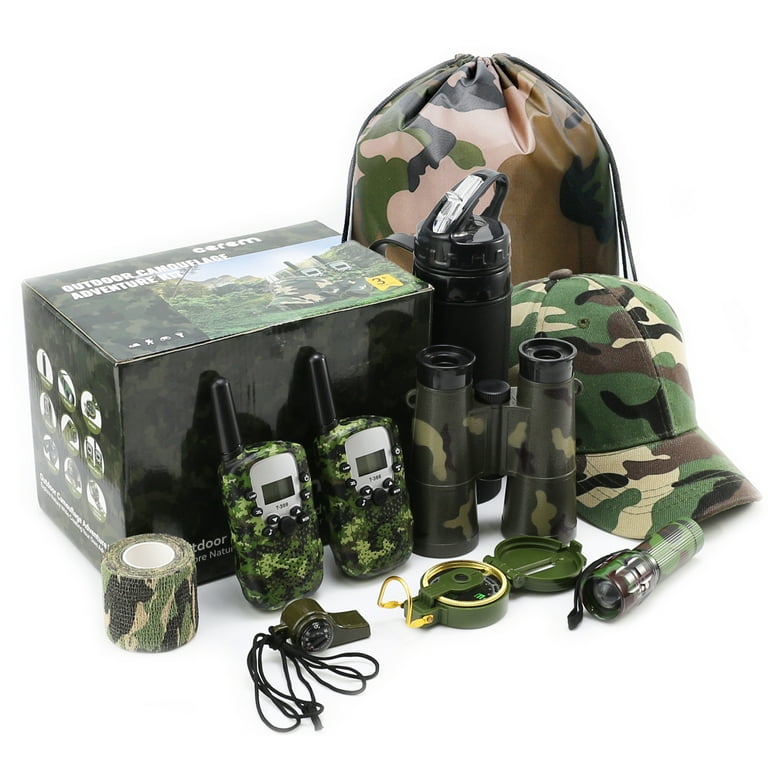The image showcases an "Outdoor Camouflage Adventure Kit" designed for children aged 3 and up. Set against a white background, the kit includes a variety of items, all predominantly featuring green, brown, tan, and black swirling camouflage patterns, except for the solid black water bottle. Prominently displayed is a camouflage ball cap and a pair of binoculars positioned on their front lenses. Nearby, two small camouflage walkie-talkies with silver-bordered screens and tiny antennas are arranged neatly. Accompanying these items are a small camouflage flashlight with a black wrist loop and a green compass with a gold rim and latch. A dark green whistle with a black string is laid out in front, and what appears to be camouflage kinesiology tape or an ace bandage is also included. All these items are gathered around a box labeling them as the "Outdoor Camouflage Adventure Kit", indicating its intended for young adventurers. The kit comes with a camouflage drawstring bag, likely used for convenient carrying and storage of all the items.